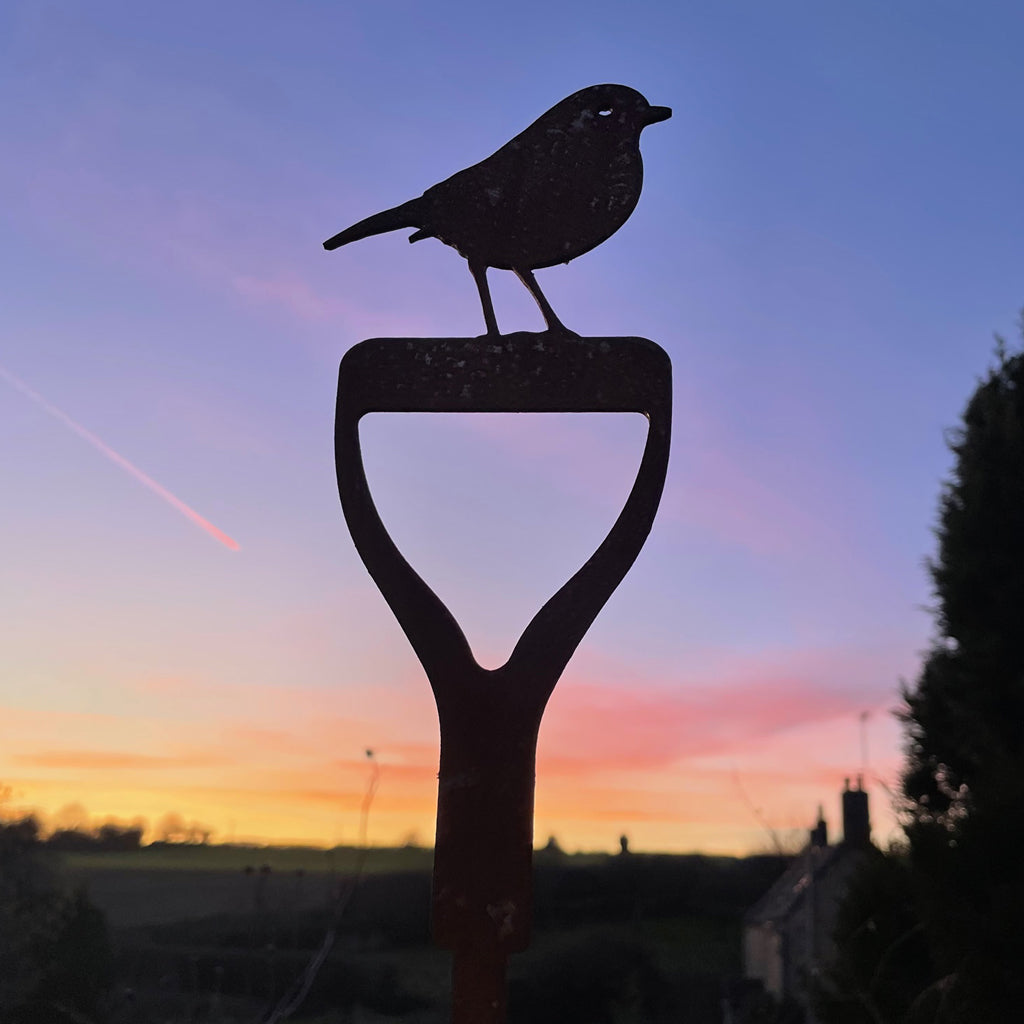The photograph, digitally enhanced and taken just after sunset or before dawn, showcases a tranquil outdoor scene dominated by a vivid sky transitioning from a deep orange at the horizon to purples and reds higher up, with streaks of pink and possibly a jet's contrail cutting through the sky. Central to the composition is the silhouette of a shovel handle sticking straight up from the ground, with a small bird perched on top. The bird, mostly in shadow except for a faint blue glint where an eye would be, faces right with its tail to the left. In the lower right corner, also in shadow, stand a tall evergreen tree and a house featuring a prominent chimney. The scene captures the serene beauty and stillness of either dusk or dawn, with a richly colored sky and defined silhouettes.